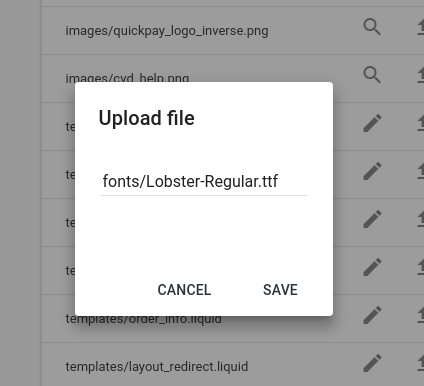In the image, a central pop-up window overlays a grayed-out background. The background consists of a square box divided into 8 rows with faintly readable text labels such as "image," "quick pay," "logo," "inverse," "ping," "image," "CBD," "help," and "ping." 

The white pop-up prominently displays the title "Upload File" in black font at the top. Below this title, the filepath "fonts\Lobster-Regular.TTF" is shown. A gray line separates the title from the actions below, where bold black text features the buttons "Cancel" and "Save." Further down, another filepath reads "templates\order_info.liquid."

On the right-hand side of the image, a vertical toolbar includes multiple icons: two magnifying glasses followed by a series of six pencil icons. The left-hand side of the top section remains empty, providing a clean contrast to the more detailed right side.